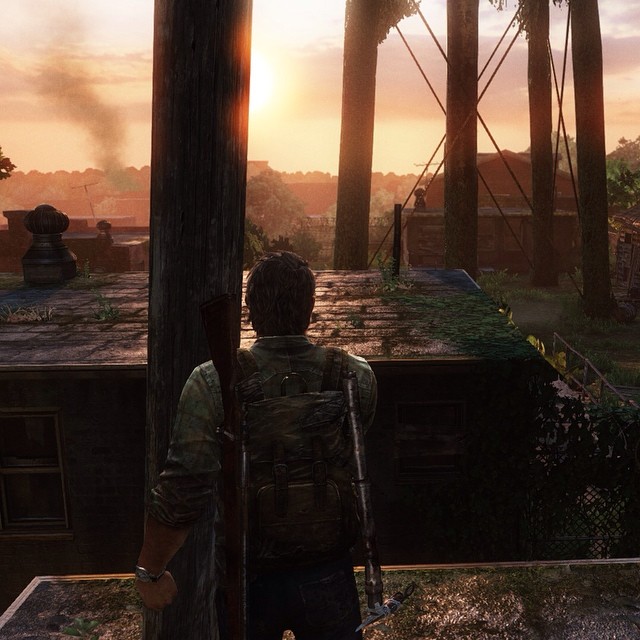In this compelling image, a man is captured standing atop a building, gazing away from the camera. His back is prominently featured, showcasing his gray, long-sleeved shirt with sleeves rolled up to the elbows. His left arm rests naturally by his side, with his hand clenched into a fist and adorned with a watch. Contrastingly, his right arm is positioned more towards the front. He carries a backpack, from which a rifle is slung over his left shoulder, while a metallic rod rests on his right shoulder. Framing the scene are a telephone pole and an adjacent building, further accentuating the urban environment in which he stands.